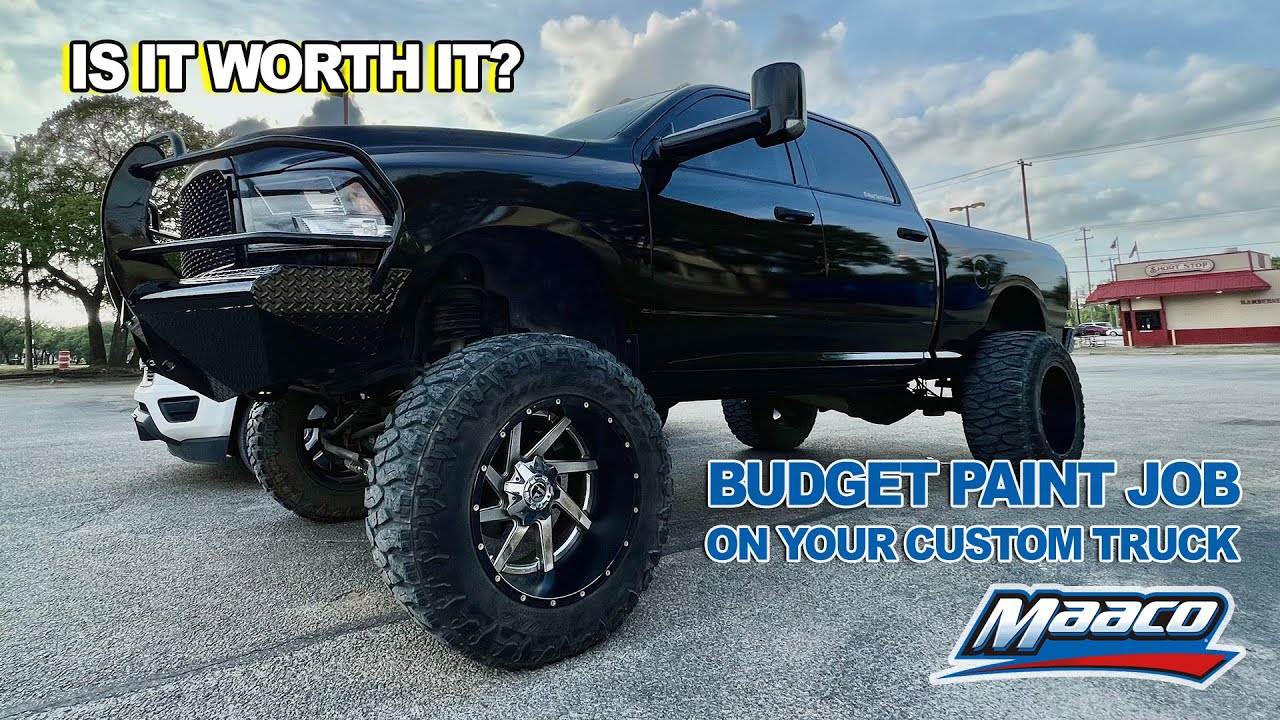The image is a full-color advertisement for MAACO, featuring their logo in red, white, and blue with white lettering and a blue and red stripe underneath. The text prominently reads "Is it worth it?" in the upper left corner, and "Budget paint job on your custom truck" in the lower right corner. The subject of the photograph is a large, shiny black pickup truck equipped with custom rims, a custom nose guard, extended side-view mirrors, and silver hubcaps. The truck, which appears to be designed for off-road purposes, is parked in a lot with a restaurant or shop that has a sign reading "Short Stop" partially visible in the background. A white car's hood and grille partially peek out from behind the truck. The scene is set on a paved parking lot under a blue sky with some clouds, and there are a few trees visible in the background.